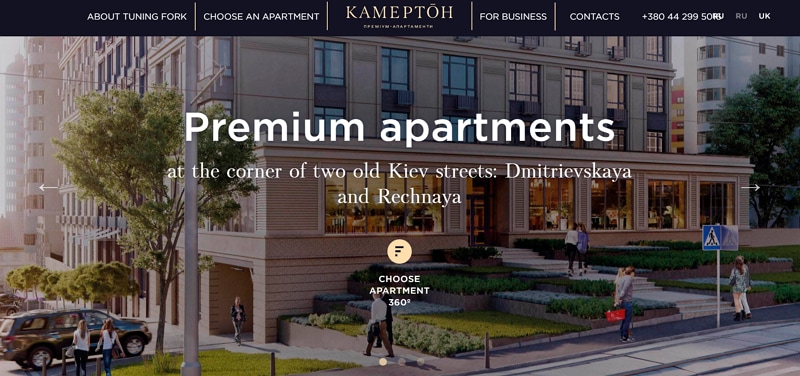A detailed caption for the image:

"Premium apartments located at the intersection of Dmitrievskaya Street and Rechnaya Street in downtown Kiev. The modern building, marked with contact information including 'KAM' and a phone number '+30 38044 29950,' stands prominently at the crossroads of these historic streets. The scene depicts a bustling urban setting with a few pedestrians: two women walking together, another woman near the parking garage, and a group near the entrance consisting of a man, a woman, a young girl, and a young boy. The vibrant street life adds a lively touch to the sophisticated atmosphere of the upscale residential complex."